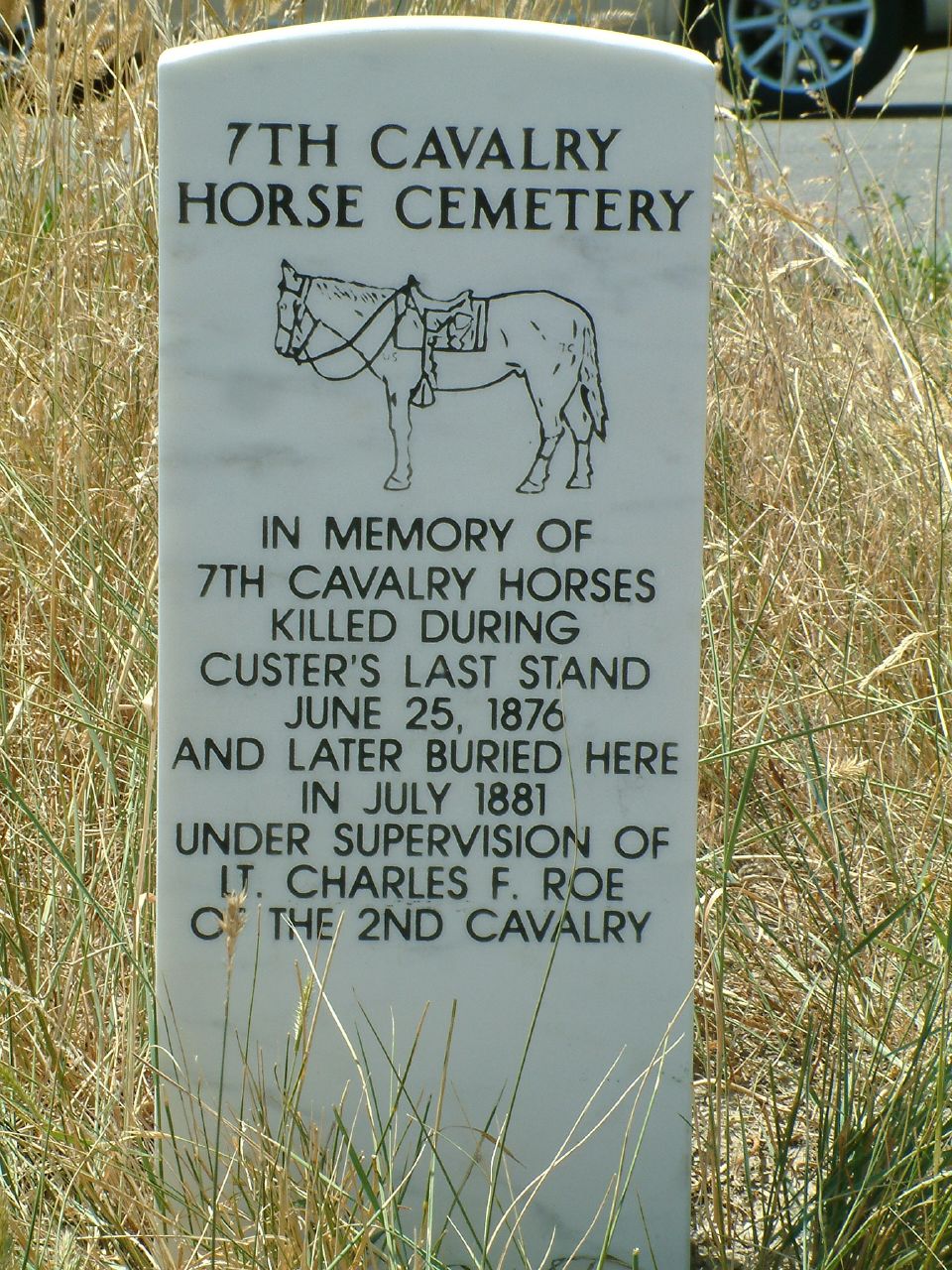The image depicts a tall, white marble tombstone situated in a field with yellow and brown grass. The tombstone, inscribed with black lettering, reads "7th Cavalry Horse Cemetery." Below this inscription, there is an illustration of a horse. Further down, the text commemorates the horses of the 7th Cavalry, noting that they were killed during Custer's Last Stand on June 25, 1876, and later buried at this site in July of 1881 under the supervision of Lieutenant Charles F. Rowe of the 2nd Cavalry. Surrounding the tombstone, grass and weeds are evident, and in the upper right corner of the image, a car tire in an adjacent parking lot is visible.